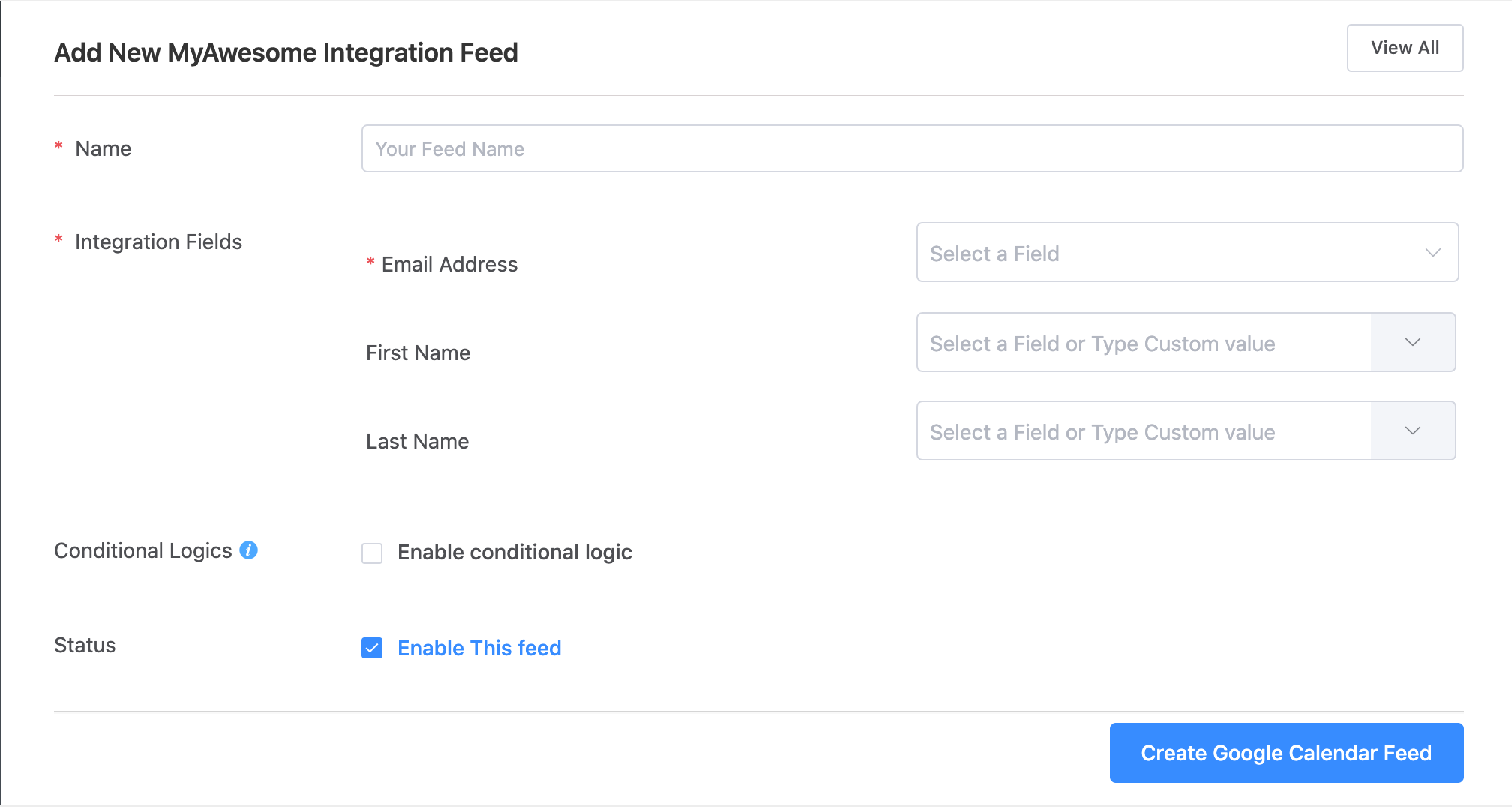This image is a screenshot of a form interface. At the top left, there is a button labeled "Add New", followed by the title "My Awesome Integration Feed" in bold black text. The form's background is entirely white. On the far right, there is a "View All" button enclosed in a box, and a horizontal line divider is situated beneath this section.

Below the top section, the form includes fields for user input. The first field is labeled "Name" with a red asterisk indicating it is a required field. The red asterisk is also accompanied by the note "integration fields". Following this, there are three fields: the first is for "Email Address" (marked with a red asterisk and currently empty), the second is for "First Name", and the third is for "Last Name".